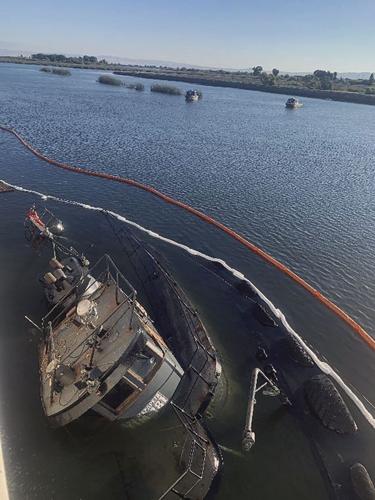In this detailed image, a capsized ship, potentially a shrimping trawler, lies tilted sideways in a river. The vessel is almost completely submerged, with parts of its multi-leveled structure including the metal railings and the bridge - now extensively rusted - peeking above the waterline. A white upper deck and lights indicate where the captain's station used to be. Surrounding the shipwreck is a yellow fence, and running parallel to it are two barriers - a white one and a red one, likely preventing the spread of pollutants such as oil. Small boats, possibly tugboats, float beyond the barriers amidst a backdrop of reeds and distant land. A crystal blue sky stretches beyond the serene yet windy water, which shows signs of light ripples. There are additional trees and more boats along the far bank, adding to the scene of recovery and containment efforts.